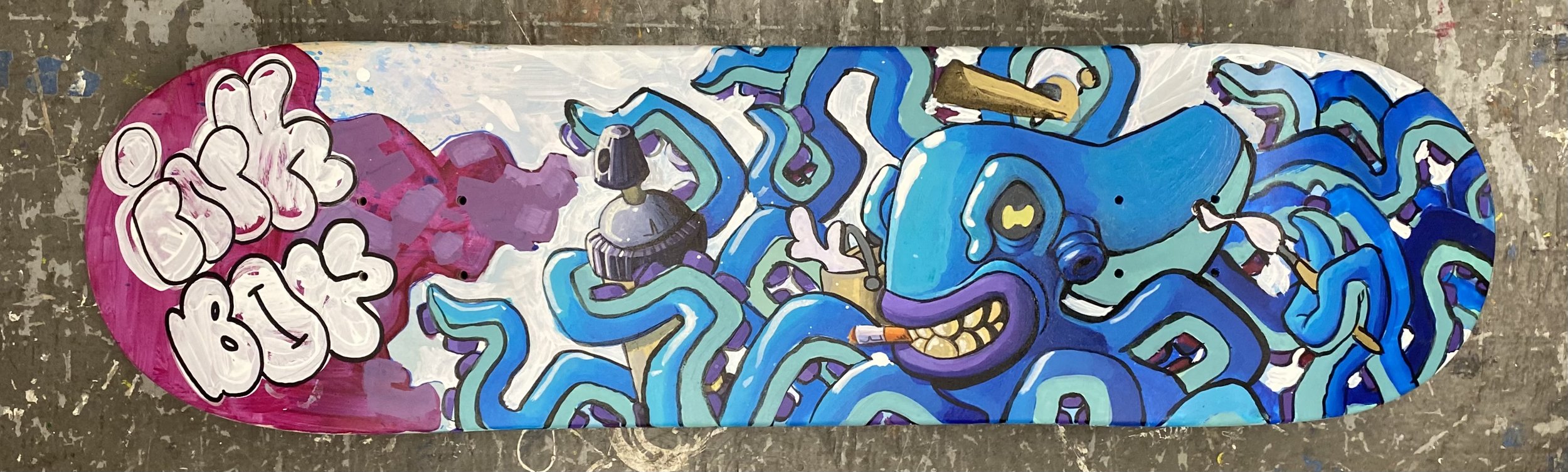The photograph showcases the underside of a skateboard adorned with elaborate graffiti-style artwork. Resting on a paint-splattered and scuffed concrete surface that exudes a worn, urban aesthetic, the skateboard becomes a canvas for street art creativity. The focal point of the artwork is a vividly detailed octopus character, depicted in shades of blue and green. With its long, sinuous tentacles extending dynamically across the deck, the octopus’s mouth is open, revealing sharp teeth, and it clutches a cigarette between its teeth. One of its tentacles grasps a can of spray paint, actively creating graffiti in vibrant purples and reds. The overall composition fuses marine imagery with urban grit, capturing the rebellious spirit of street art.